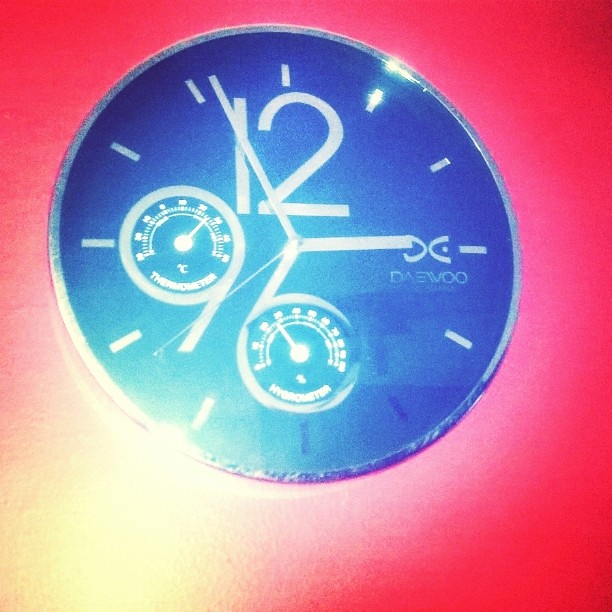The image features a close-up shot of a wall-mounted timepiece with additional measurement gauges. The primary feature is a central clock marked prominently with a large '12' at the top, but no other numerical indicators, only hash marks. Surrounding the clock face are two additional measuring instruments: a thermometer on the left, calibrated in degrees Celsius, and a hygrometer at the bottom, designed to measure humidity. The background of the clock face appears to be a gradient that shifts from blue to black. The entire setup is set against a vivid red background. The Daewoo logo is visible on the timepiece, albeit the exact spelling is somewhat obscured. The photo quality is grainy and affected by a bright flash originating from the bottom left corner, which has caused a yellowish bleaching effect over that part of the image.